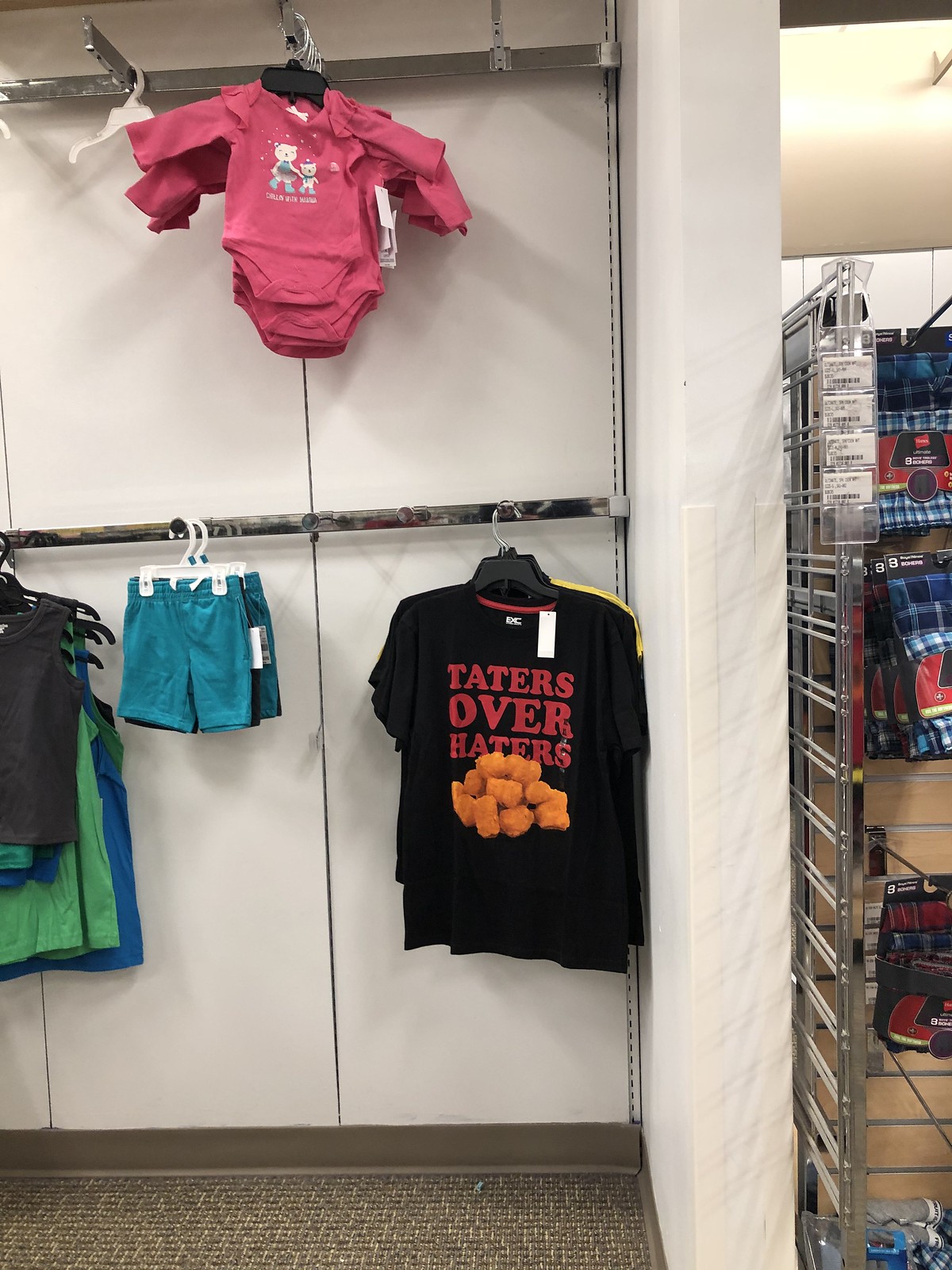The image depicts a brightly lit children's clothing section within a store, featuring white walls and a grey patterned floor. On the left two-thirds of the image, there are two main racks. The top rack, approximately six feet off the ground, displays pink baby onesies adorned with a cartoon of a mama bear and child bear, with a snowy background and unclear text. Beneath these, a medium-height rack about four feet off the ground holds various clothing items on hangers. Prominently, there is a black t-shirt with the phrase "Taters over Haters" and imagery of tater tots, flanked by little boys' pants in blue and green, likely for two to three-year-olds. Beside these are additional hangers showcasing blue, green, and black tops against the white wall. On the right side, a wire display rack is partially visible, holding items that may be socks or underwear, with indistinct colorful prints in blues, reds, and oranges. A white divider marks the transition from this section to the rest of the store in the background.